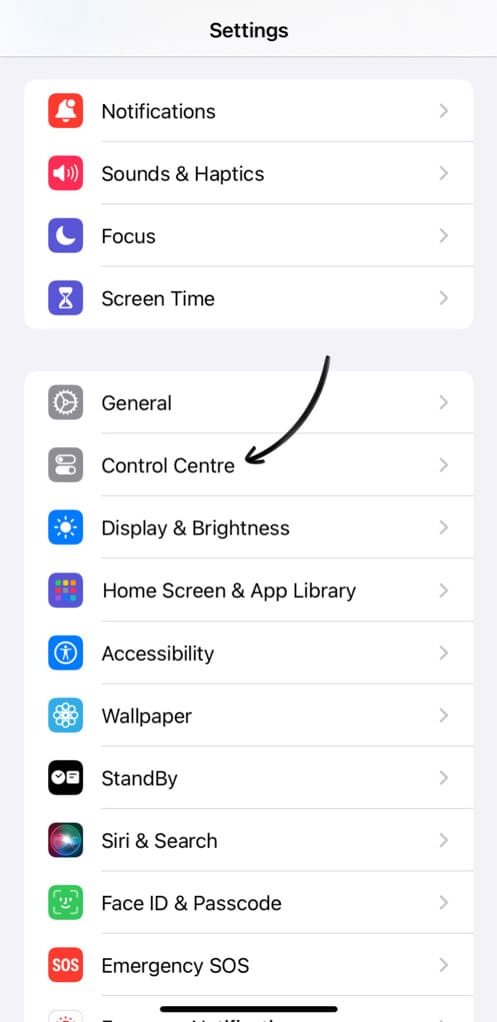This image is a screenshot of the "Settings" menu on an iPhone, featuring various tabs and their corresponding icons. 

1. **Notifications** - Displayed at the top with a red icon.
2. **Sounds & Haptics** - Marked by a pinkish icon.
3. **Focus** - Identified with a purple icon.
4. **Screen Time** - Also has a purplish icon.
5. **General** - Features a gray gear icon.
6. **Control Center** - Illustrated with a gray icon.
7. **Display & Brightness** - Characterized by a blue icon.
8. **Home Screen & App Library** - Marked with a purple icon.
9. **Accessibility** - Has a blue icon featuring a person inside a circle.
10. **Wallpaper** - Displayed with a light blue icon depicting a simplistic flower shape.
11. **Standby** - Represented by a blackish icon.
12. **Siri & Search** - Features a multicolored icon.
13. **Face ID & Passcode** - Identified with a green icon with a face shape.
14. **Emergency SOS** - Has an orange or red icon with the letters "SOS" inside.

Additionally, there's a black arrow pointing in a curved manner towards the "Control Center" tab, highlighting it specifically.